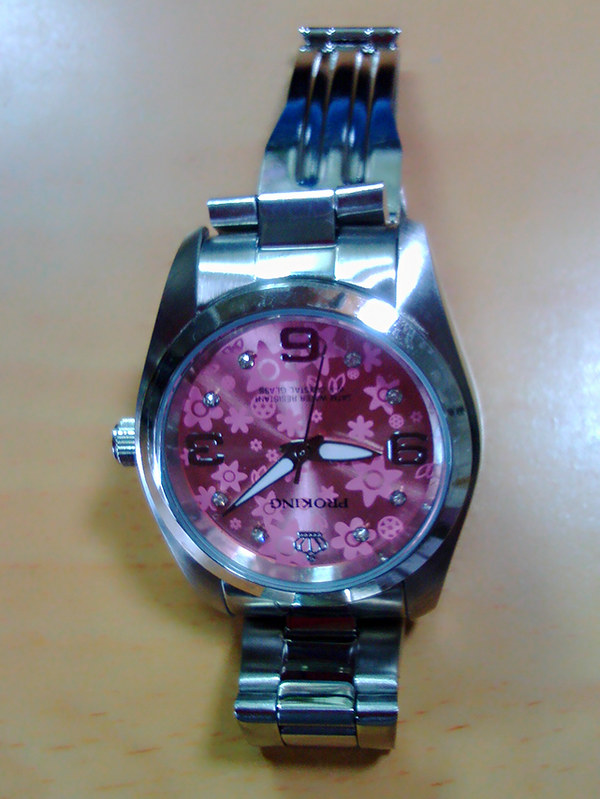The image is a vertically rectangular frame featuring a wristwatch viewed from above. The wristwatch is oriented upside down, with the 12 o'clock position at the bottom of the frame and the 6 o'clock at the top. The watch band is silver, complementing the dark pink dial adorned with lighter pink floral patterns. The dial displays only the numbers 3, 6, and 9, with the 12 o'clock position marked by a small silver crown. The remaining hours are indicated by simple silver dots. The watch has white hour and minute hands and a black second hand, offering a striking contrast against the vibrant pink background.